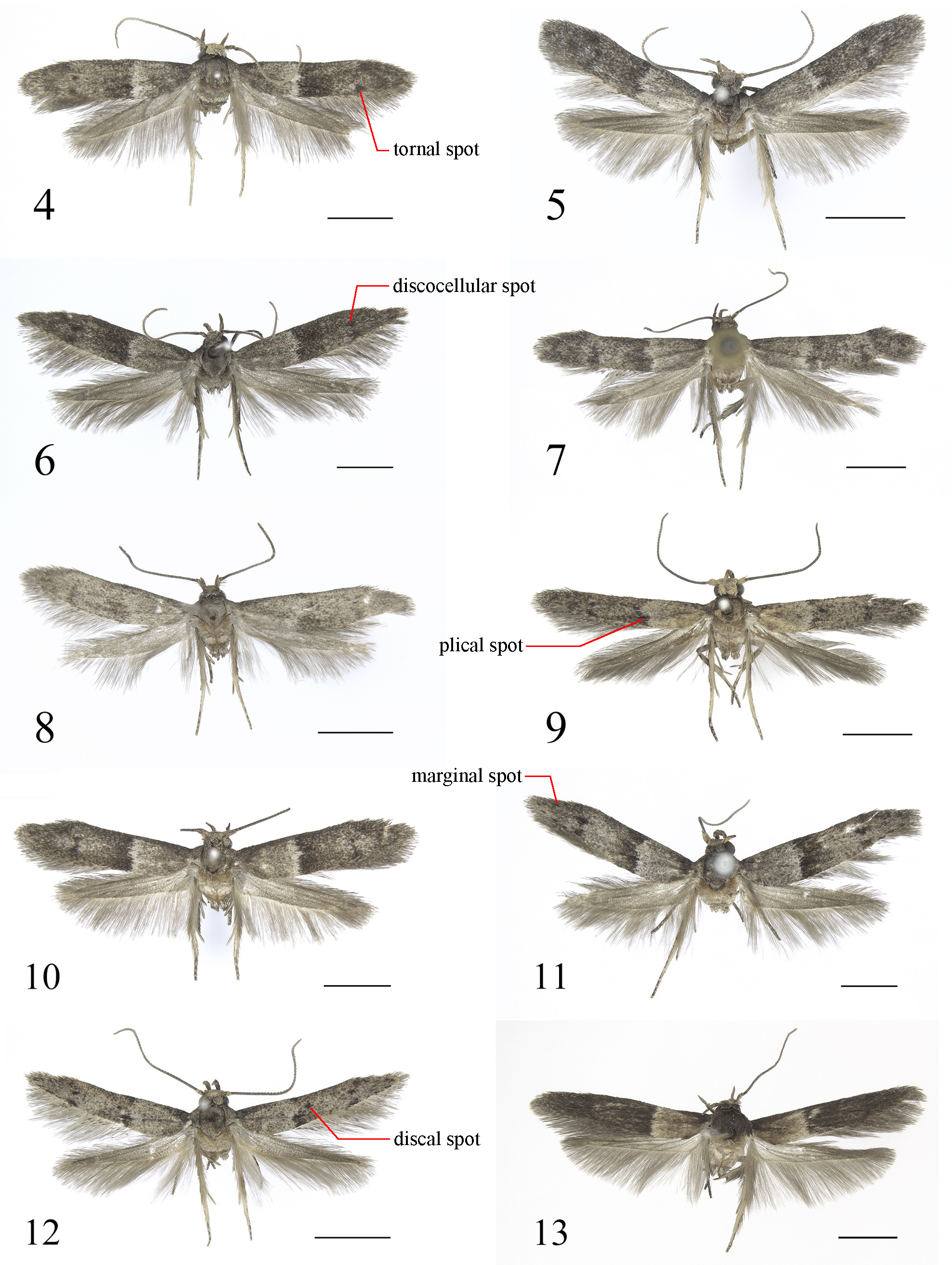The informational chart features a vertically aligned rectangular image showcasing a series of images of what appears to be the same species of gray moth-like insect. There are 13 numbered images in total, beginning with number 4 and ending with number 13, arranged in two columns of five rows each. The left column consists of images 4, 6, 8, 10, and 12, while the right column includes images 5, 7, 9, 11, and 13.

Each insect is depicted with its wings spread, revealing distinct variations and positions. Starting from the top left, image number 4 displays a gray moth with filament-covered wings and two antennae, marked with a red arrow indicating a "tornal spot" on its wing. Image number 5 shows the same moth in a slightly different position with its wings more widely spread.

Image number 6 highlights the "discocellular spot" on the moth’s wing with a red line. Number 7, like previous images, presents the moth with its wings spread even further. Number 8 shows a moth of the same species but with noticeably smaller wings.

Further down, specific wing parts are labeled with red lines: number 9 indicates the "plical spot," number 11 focuses on the "marginal spot," and number 12 highlights the "discal spot." The insects are set against a clean white background, emphasizing the detailed spots and patterns on their wings.